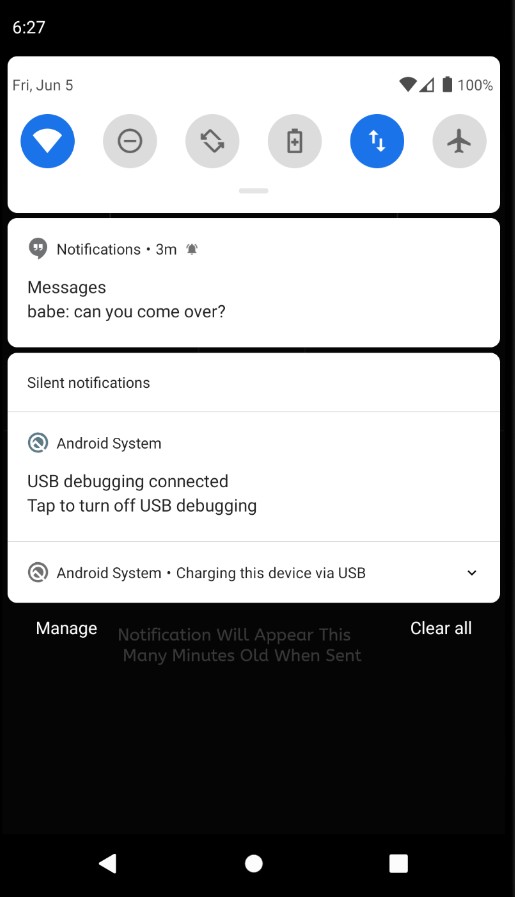The screenshot taken from a smartphone displays a predominantly black background with three distinct white rectangular sections. 

At the top of the screen, the first white section indicates the date "Friday, June 5th" on the left and shows a status bar in the upper right corner. The status bar includes a Wi-Fi signal icon with minimal bars, a 100% battery indicator, and other icons. From left to right, these icons are: an active blue Wi-Fi symbol, a gray "Do Not Disturb" icon, a gray "Rotate Screen" button, a grayed-out battery icon, a blue circle with an up-and-down white arrow indicating some type of connectivity, and a grayed-out airplane mode button.

The middle white section displays notifications. The first notification, received three minutes ago, is from "Messages" with the text "Babe, can you come over?" Below that, in this same section, an Android system notification states "Silent Notifications." Further details specify "USB debugging connected" with an invitation to "Tap to turn off USB debugging" and "Charging this device via USB."

The bottom white section transitions into the black background, featuring faded gray text that reads, "Notifications will appear this many minutes old when sent." To the right in white, the option to "Clear all" notifications is available, while "Manage" appears to the left. At the very bottom of the screen, there are three horizontally aligned white icons, but their specific details are not provided.